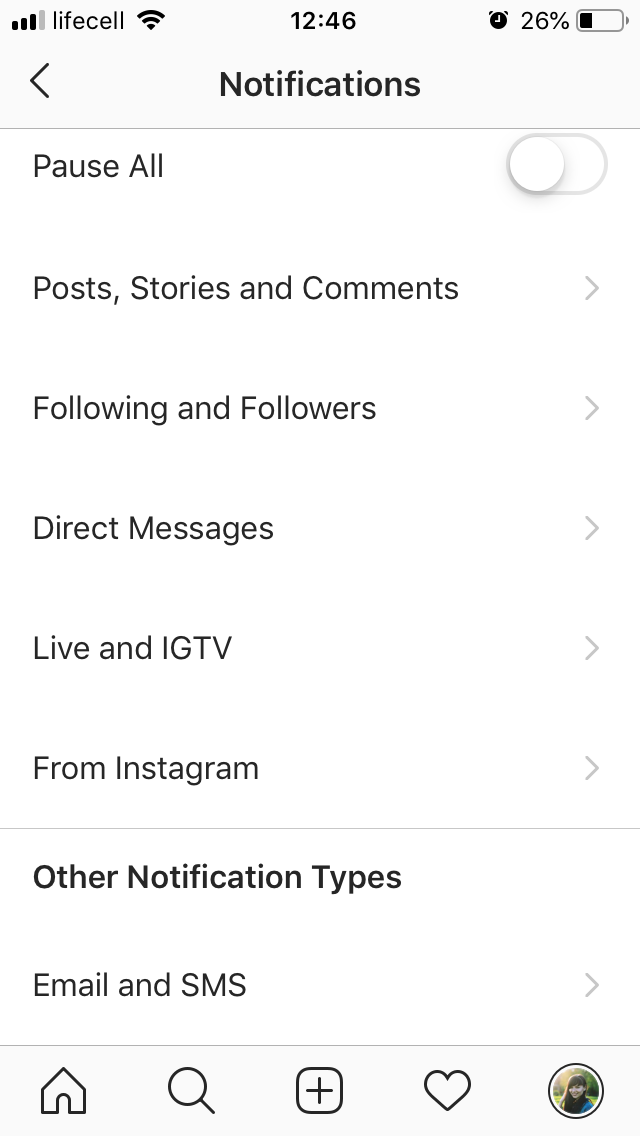The image showcases a smartphone screen featuring numerous interface elements of an Instagram application. At the top of the screen, the status bar displays the signal strength with three out of four bars, alongside a 'Life Cell' carrier label, and the Wi-Fi icon. The time is shown as 12:46 PM and the battery level is at 26%.

Below the status bar, the screen includes a series of settings starting with a bar labeled "Notifications" prefaced by a less-than symbol (<). Directly beneath this, the "Pause All" option is displayed alongside a toggle switch set to the left. Subsequent options include "Post Stories and Comments," "Following and Followers," and "Direct Messages," each associated with its respective functions.

Further down, the interface highlights sections labeled "Live" and "IG TV," followed by "From Instagram." A horizontal line separates these options from another category labeled "Other Notification Types" where "Email and SMS" notifications are listed. Each of these lines ends with a greater-than symbol (>), indicating that they can be expanded for further details.

At the bottom of the screen, a navigational bar contains five primary icons: the home icon for returning to the main feed, a magnifying glass for searching, a square with a plus symbol for creating new posts, a heart icon for checking likes and interactions, and a profile picture for accessing the user's profile.